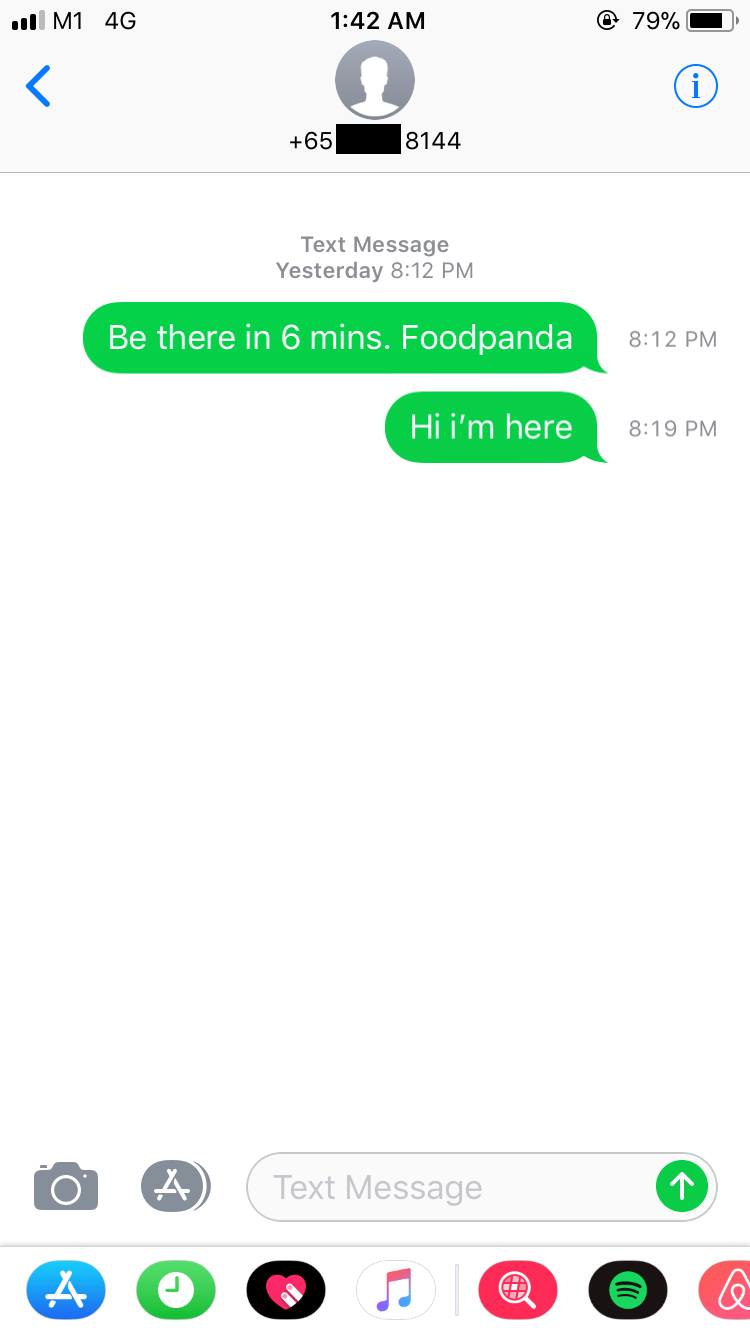This is a detailed screenshot of a text message conversation on a person's cell phone captured at 1:42 AM, as indicated at the top right corner. The phone has three bars of network coverage displaying "M1 4G," and the battery stands at 79% capacity. The contact's phone number starts with "+65" but is partially obscured except for "8144" due to blacked-out information for privacy.

In the conversation, both messages are timestamped from the previous evening, beginning at 8:12 PM with a text saying, "Be there in six minutes, food panda." The following message, sent at 8:19 PM, reads, "Hi, I'm here." Both messages appear in green text bubbles with white text, indicating they were sent from the phone being used.

At the bottom section of the screen, there are several interface elements visible, including the camera and app store icons, the message composition bar, and the send button (a green circle with a white upward-pointing arrow).

The dock shows a blue icon with a white 'A' (likely the App Store), a green icon with a white clock face, a black icon with a red heart (possibly for health-related applications), a white icon with a musical note (likely the Music app), a red icon with a white magnifying glass (probably a search app), a green icon for Spotify, and a red icon for Airbnb.

No people or animals are depicted in this image, focusing solely on the digital conversation and user interface of the mobile device.